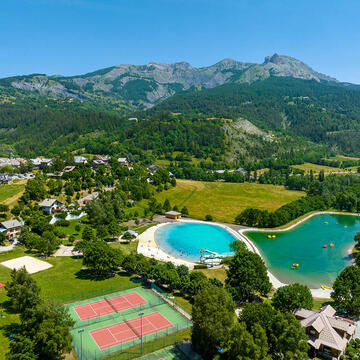This aerial image, likely captured by a drone, showcases a picturesque resort or country club nestled in a lush, mountainous region. Central to the scene are two prominent tennis courts with burgundy-colored clay surfaces, surrounded by green areas and fencing. The courts are bordered by lines of trees on the left and right, with taller trees behind them, overshadowing a small home with a beige roof. To the right of the courts lies a vast green clearing lined with trees and shrubbery.

Adding to the resort's natural beauty are two distinct bodies of water. The first is a custom-made, oval-shaped pool with brilliant cyan water, encircled by sandy white soil, giving it a beach-like appearance. The second body of water is a more natural-looking pond with deep aqua-green water, home to several small yellow paddle boats floating across its surface. This pond is also surrounded by a narrower sandy edge.

In the distance, the scene is framed by towering gray mountains and rolling hills dotted with a diverse array of trees, from lush forest varieties to firs and pines. The bright daylight enhances the vivid colors and natural beauty of the landscape. A housing development is visible in the left-hand portion of the image, along with a small orange shack with a beige roof near the ponds, adding further intrigue to this scenic, well-maintained community.